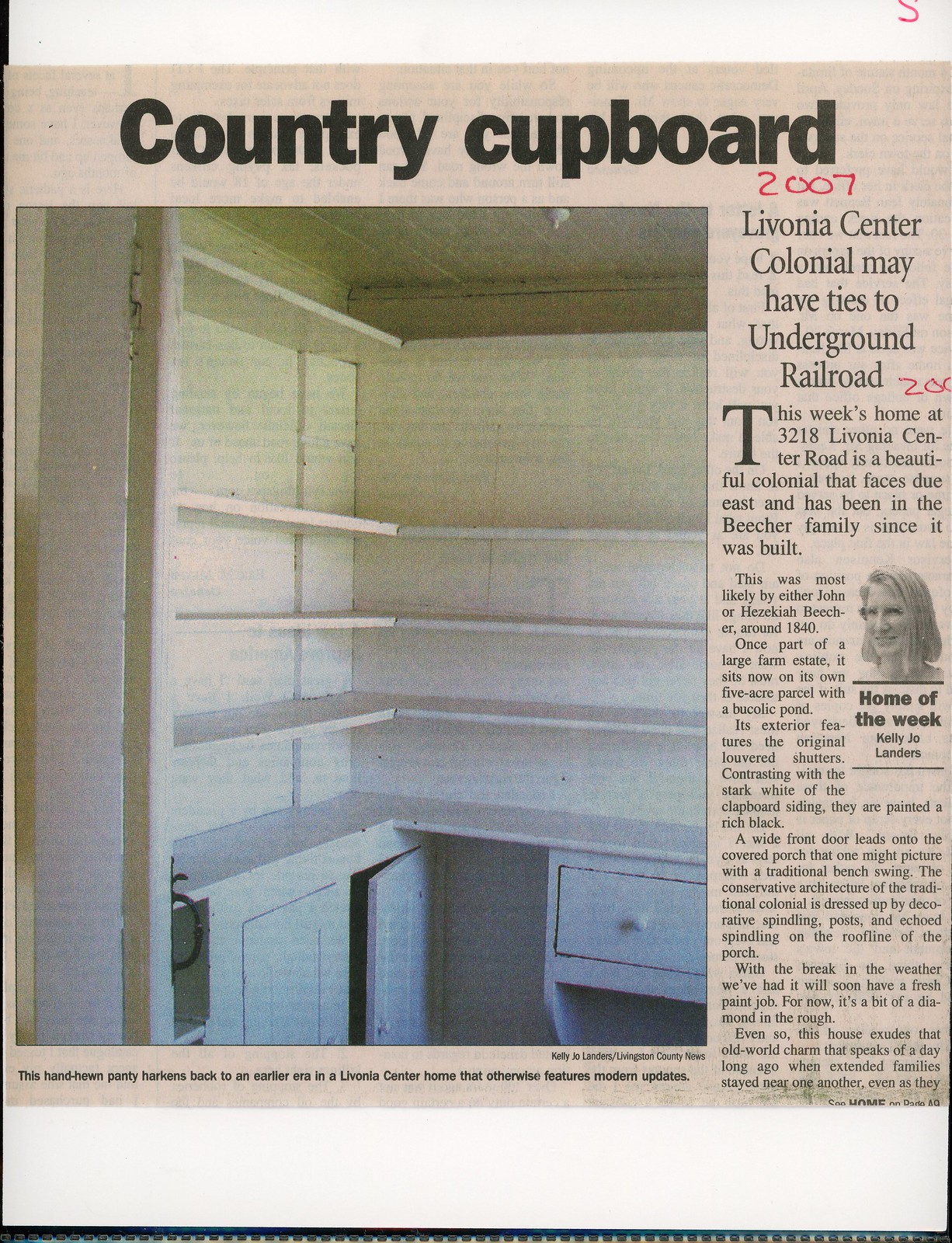The photograph displays a cutout of an old newspaper article. The cutout, set against a light peach background with a white sheet of paper on top, is headlined in bold black font: "Country Cupboard." Notably, the handwritten note "2007" is inscribed in red ink on the right-hand side of the header. The subheading, "Livonia Center Colonial May Have Ties to Underground Railroad," introduces the article below. A hand-penned "S" and the number "200" also appear in red ink around the article. 

The article describes a historic home located at 3218 Livonia Center Road, a beautiful colonial facing due east, which has remained in the Beecher family since its construction, likely around 1840 by either John or Hayes K. Beecher. Originally part of a large estate, the home now sits on a five-acre parcel featuring a serene pond. The exterior is characterized by original louvered shutters painted black, contrasting with the stark white clapboard siding, and a white front door leading to a covered porch adorned with decorative posts and spandrels typical of traditional colonial architecture. The house, while in need of some fresh paint, maintains a quaint old-world charm reminiscent of a time when extended families lived nearby.

On the right side of the newspaper clipping, a small black-and-white photograph of the article's author, Kelly Jo Landis, is placed. She is identified in the caption "Home of the Week," and the accompanying photo shows her with short hair and glasses. The left side features a full-page image of an indoor pantry room, notable for its hand-hewn wooden cabinets and shelves, which recalls an earlier era even in a modernized Livonia Center home. The caption below the pantry image reads, "This hand-hewn pantry harkens back to an earlier era in a Livonia Center home that otherwise features modern updates." The article appears to continue on page 49.